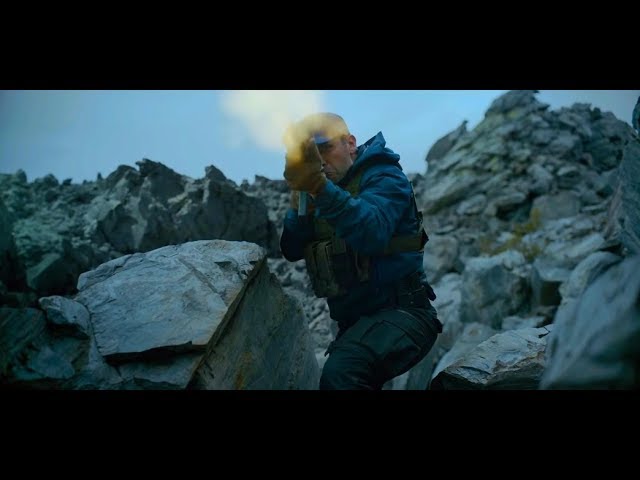This is a horizontally rectangular photograph framed by thick black borders at the top and bottom. The image depicts a man standing in a rugged, mountainous area with jagged gray and black rocks. The environment has patches of lighter color, possibly moss or lichen. He is pictured mainly from the knees up, somewhat facing forward with his front knee slightly bent. The man appears heavily equipped, wearing dark gray cargo pants with a green tactical belt and harness, both adorned with multiple pouches and tools. His upper body is clad in a dark jacket, possibly resembling a puffer jacket with a hood, and a blue hoodie underneath with the hood down. His hands, covered in tan gloves, are positioned near his head, one possibly holding a machine gun while firing, and he might be holding or looking at a golden object with smoke emanating from it. The background reveals a darkening sky, suggesting either sunset or dusk, adding a dramatic contrast to the bright area around his head, possibly from sunlight reflecting off a hat. The man might also be wearing glasses, enhancing the detail and mystery of this dim yet compelling scene.